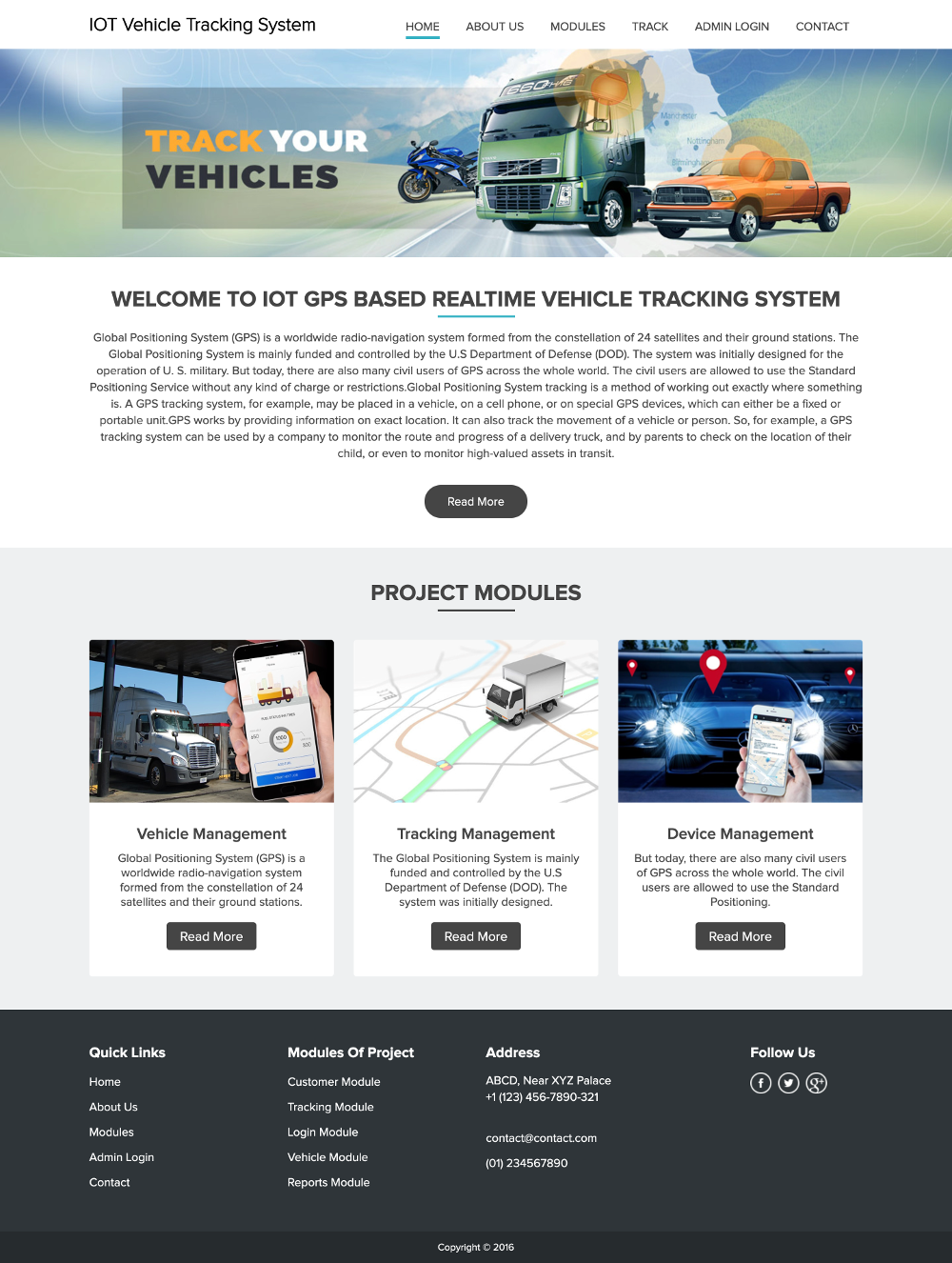This is a screenshot of a webpage that features a vehicle tracking system utilizing IoT technology. The background is predominantly white with various graphical elements and extensive text. At the top of the page, in bold black text, it reads "IoT Vehicle Tracking System." Below this heading, there is a navigation menu with several submenus, including "Home" with a blue underline, "About Us," "Modules," "Track," "Admin Login," and "Contact."

Directly underneath the navigation menu, there's an image accompanied by the text "Track Your Vehicles." The image features a variety of vehicles: a blue motorcycle, an olive green semi-truck, and an orange pickup truck. Below this visual, in black text, the page welcomes visitors with "Welcome to IoT GPS-Based Real-Time Vehicle Tracking System." There are two paragraphs of black text that are too small to be easily read, followed by a prominent black button with white text that says "Read More."

Scrolling further down, there's a gray section titled "Project Modules" in black text. The first module is "Vehicle Management," represented with an image of a semi-truck possibly at a gas station, and a hand holding a smartphone displaying an image of a gold vehicle. This module includes a paragraph of black text and a black "Read More" button.

The second module is "Tracking Management," depicted with an image of a small white box truck navigating a street marked with orange, green, purple, and blue lines. There is a paragraph of text and another "Read More" button.

The third and final module is "Device Management," illustrated with an image of sedans overlaid with a blue filter and a red location pin. A hand is holding a smartphone once again. This section also contains about a paragraph of text and a "Read More" button.

At the bottom of the page is a black section with white text listing "Quick Links," including "Home," "About Us," "Contact," "Modules of Project," and "Address." A phone number is provided alongside the invitation to follow the project on Facebook or Twitter, indicated by their respective icons. The page concludes with a copyright date at the very bottom.